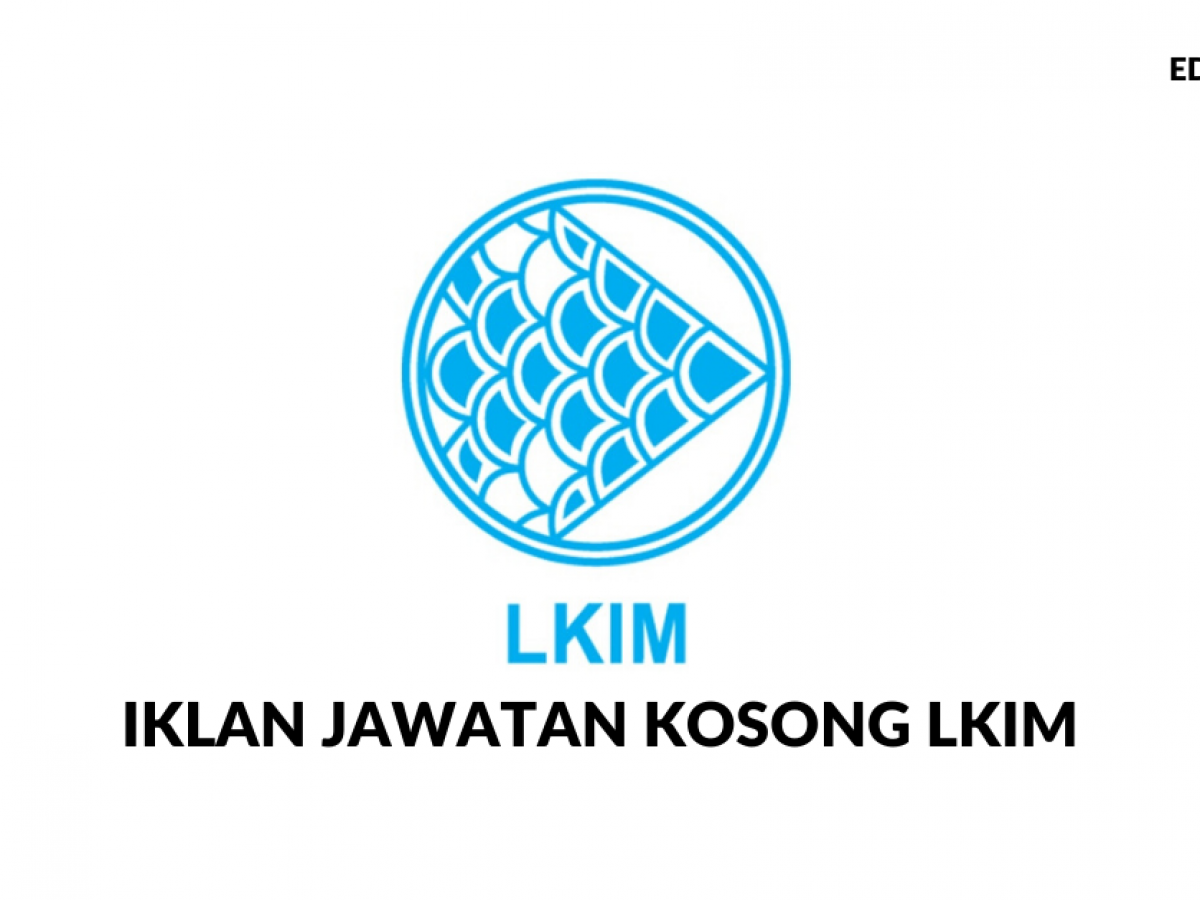The image depicts a promotional logo on a white background with black text reading "E-T" in the top right corner. Centrally, a white circle bordered by a double-lined, mid-tone blue ring encloses a unique triangular shape. This shape tapers to a point on the right, with its left side more rounded. Inside this triangle is a pattern resembling fish scales, composed of numerous blue segments bordered by white, creating a visual effect where some scales appear more filled than others. Below the circle, the acronym "L-K-I-M" is prominently printed in blue. Further below, in black capital letters, the text "IKLAN JAWATAN KOSONG LKIM" provides additional information, likely indicating the nature or affiliation of the logo.